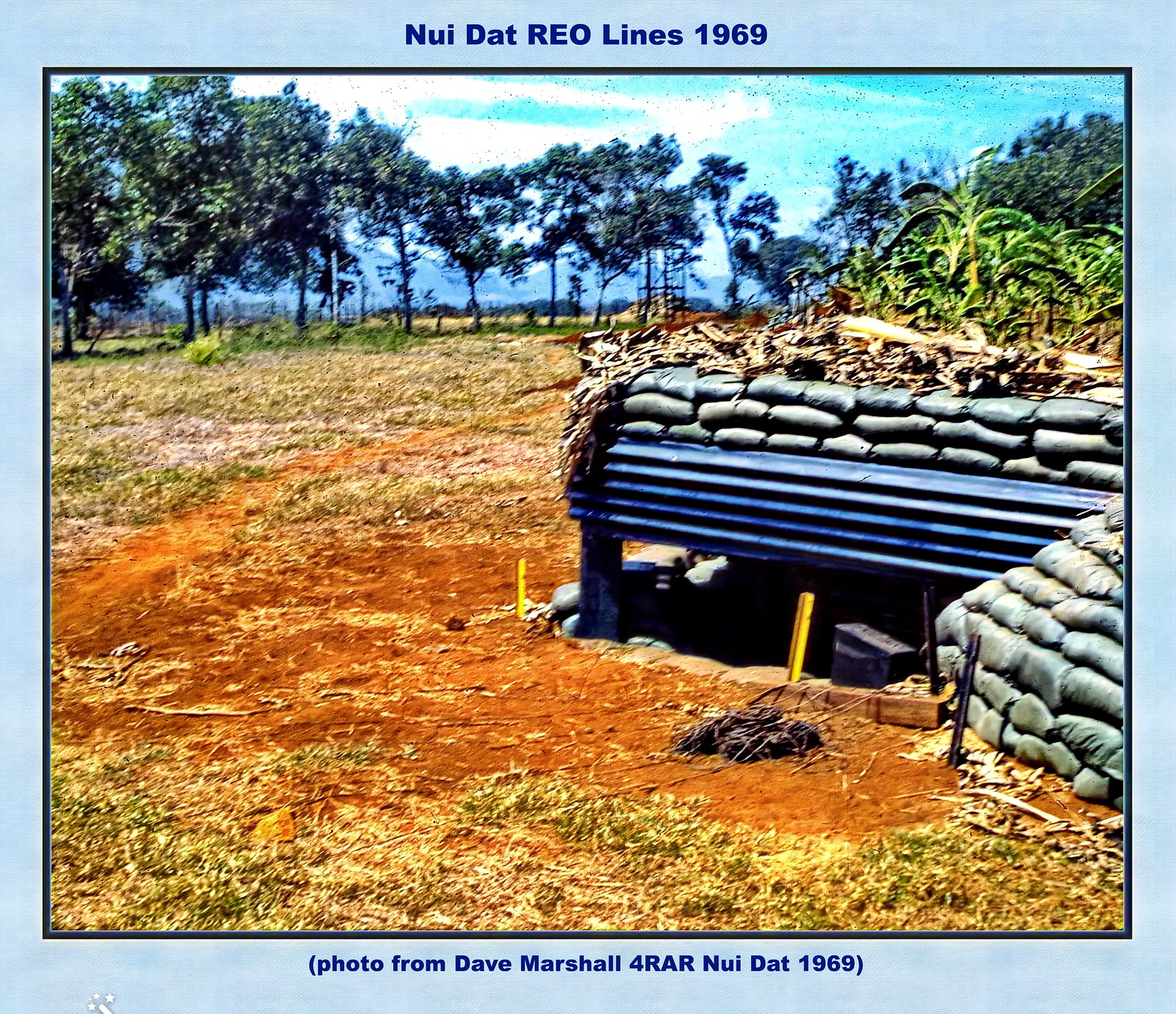"1969 photograph by Dave Marshall depicting military life in Vietnam. On the right side of the image, a series of sandbags are meticulously stacked, their hues varying between blue, gray, and brown. In front of the sandbags, a brightly colored yellow peg marks the entrance to a foxhole, which disappears into a dark and mysterious void beneath the surface. The foxhole is reinforced with a blue, ridged horizontal material acting as its roof. The surrounding terrain features rich, bright brown soil, contrasting starkly with the daylight above."